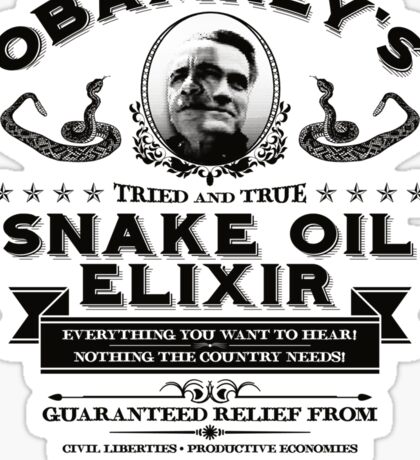The image portrays a black-and-white, old-time, satirical advertisement for "Snake Oil Elixir." The top part of the label features a partially cut-off brand name. Central to the composition is an oval-shaped portrait of two men's faces melding into each other, possibly politicians, framed by intricate illustrations of coiled snakes on either side. Above the portrait, in a banner adorned with stars on each end, are the words "Tried and True." Below this, the bold text reads "Snake Oil Elixir." A ribbon underneath proclaims "Everything you want to hear, nothing the country needs!" followed by "Guaranteed relief from civil liberties, productive economies." The overall design combines elements of line art illustration, black-and-white photography, and graphic typography, emphasizing its satirical nature.